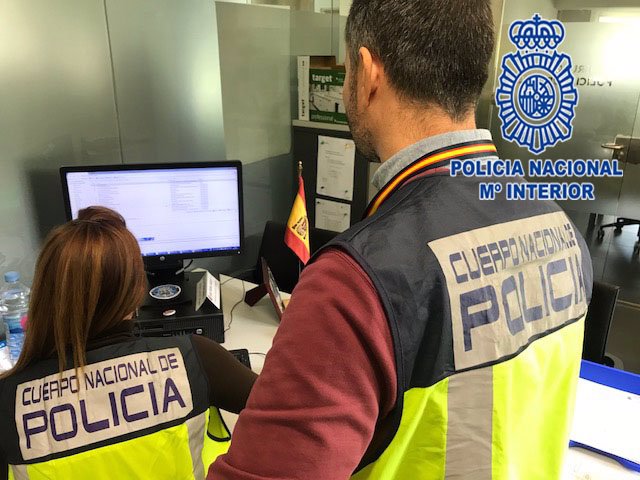This is a detailed color photograph depicting a scene within a police department. A young Latin American woman, with long hair, is seated at a white-topped desk, intently focused on a computer screen displaying indecipherable blue text. Standing closely behind her, a man, wearing a maroon shirt underneath his reflective vest, looks over her shoulder at the screen. Both are around their 30s and clad in distinctive black and yellow vests labeled "Cuerpo Nacional de Policia." In the top right corner of the frame, a blue shield adorned with a crown and additional coat of arms details signifies the "Policia Nacional," reinforcing their official capacity. The background reveals beige walls, filing cabinets, and glass doors, situating the scene clearly within a professional, bureaucratic environment. The intricately detailed logo resembles a ceremonial medal, accentuated by a blue starburst design beneath a crown, further emphasizing the formal setting of this police department.